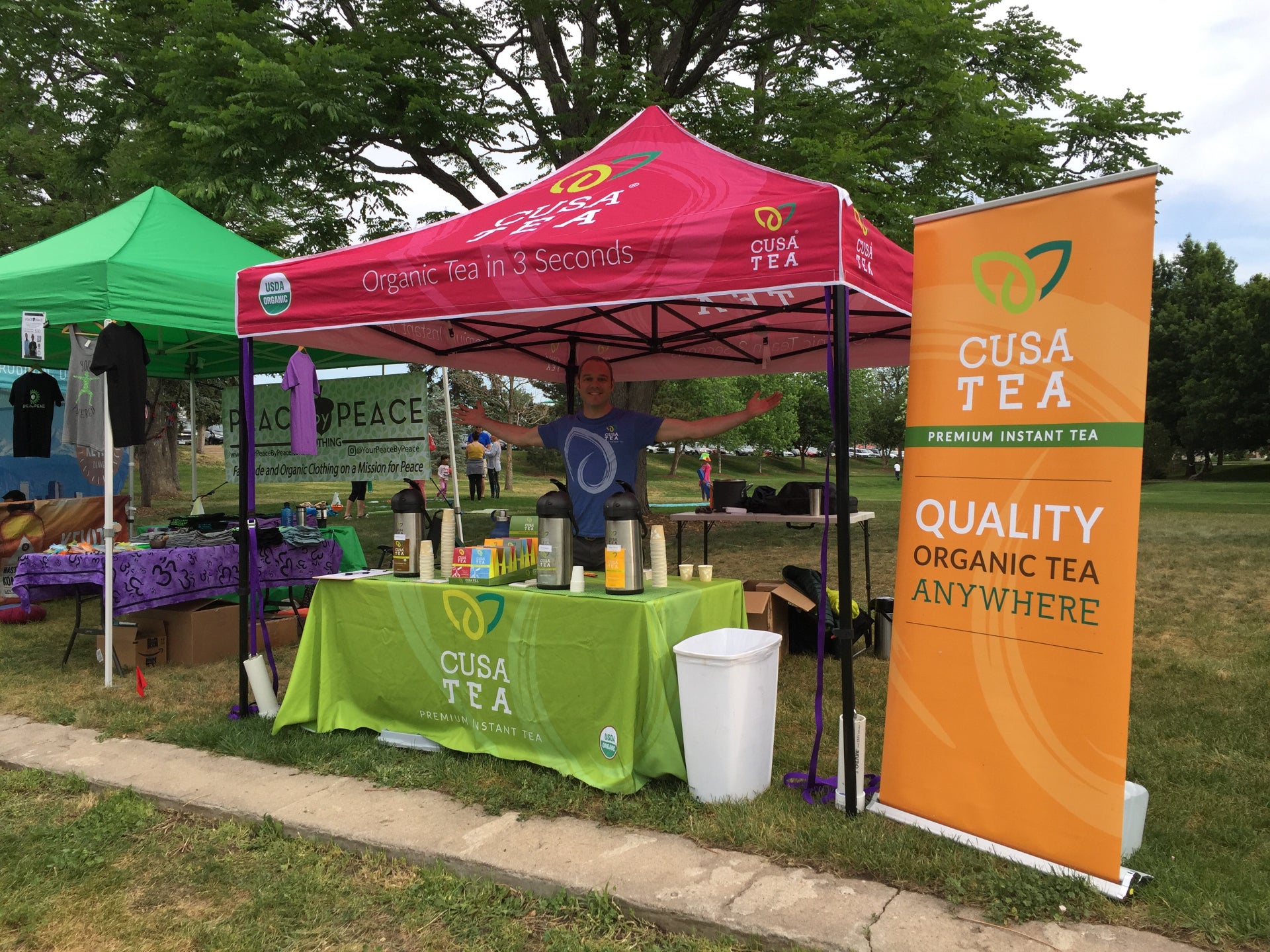In the foreground of the image, a vibrant outdoor market display captures attention. Dominating the scene is a small pavilion shelter, its hot pink awning emblazoned with the words "Cusa T," and further promoting "organic tea in three seconds." Below the pavilion, a table dressed in an olive green cloth, also marked with "Cusa T," displays a variety of tea-related items. The spread includes several tea brewing machines, an array of different-sized cups, and neatly arranged boxes presumed to be filled with tea.

Behind the table stands a white man, confidently gesturing with arms open wide. He is clad in a blue t-shirt, giving off an inviting aura. To the immediate right of this table, an upright orange banner proclaims "Cusa T," endorsing "premium instant tea, quality organic tea anywhere."

Flanking this tea stand to the left is another table, this one covered with a purple cloth and showcasing an assortment of folded clothing. Above this table is a green pavilion. Both stands are positioned on well-maintained green grass with a narrow stone sidewalk stretching in front of them. In the background, a leafy tree provides a hint of nature, suggesting the market is set in a park-like environment. The scene is drenched in a palette of colors: hot pink, olive green, sky blue, orange, and purple, creating a visually engaging and lively atmosphere.